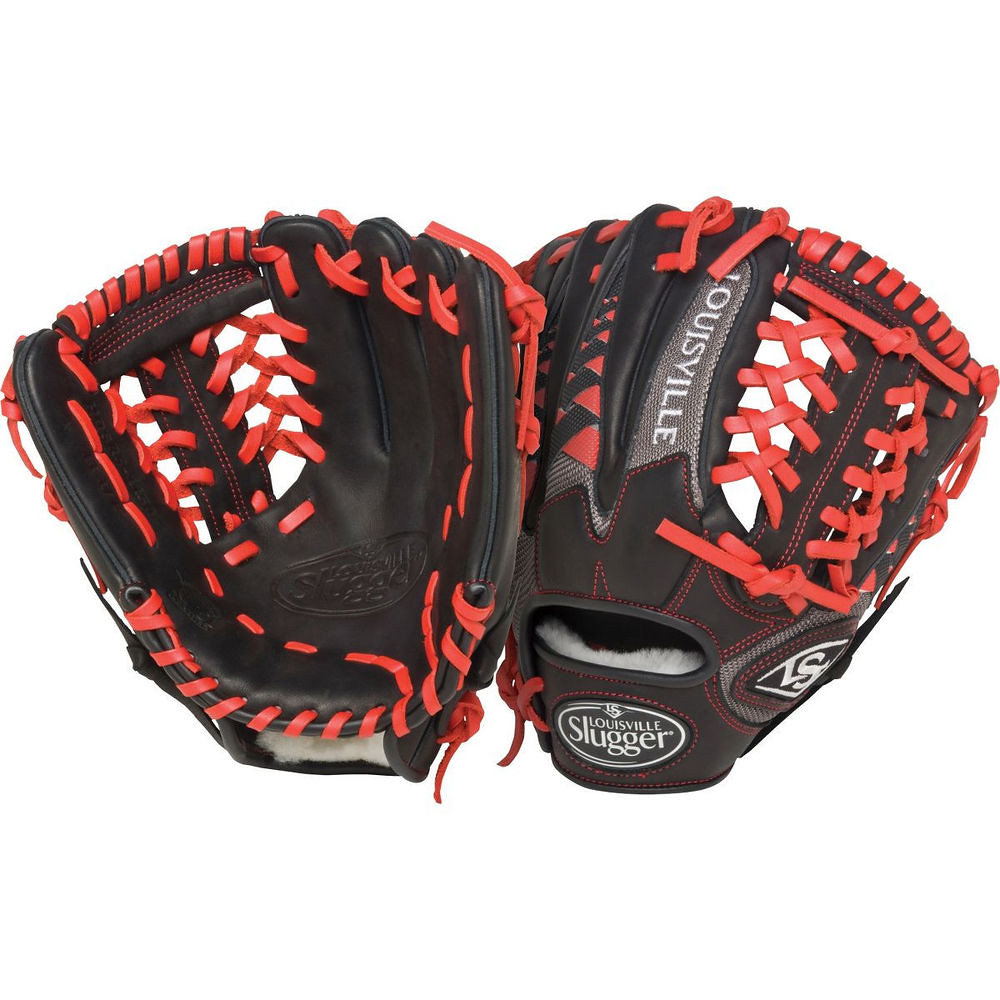This is a high-quality product photograph of two Louisville Slugger baseball gloves, reminiscent of an advertisement. The background is a clean, plain white, emphasizing the gloves. Both gloves are crafted from black leather with prominent red lacing throughout. The left glove has its palm facing the camera, showcasing the embossed "Louisville Slugger" logo on the palm and detailed, neat stitching. The glove on the right, slightly overlapping the left, displays the back of the mitt. The right glove features white "Louisville Slugger" lettering at the wrist, with the "LS" logo in gray just above it. The middle finger of this glove also has "Louisville" stitched in gray. The interior lining of the gloves appears soft, providing added comfort. The overall presentation highlights the superior quality and craftsmanship of Louisville Slugger gloves.